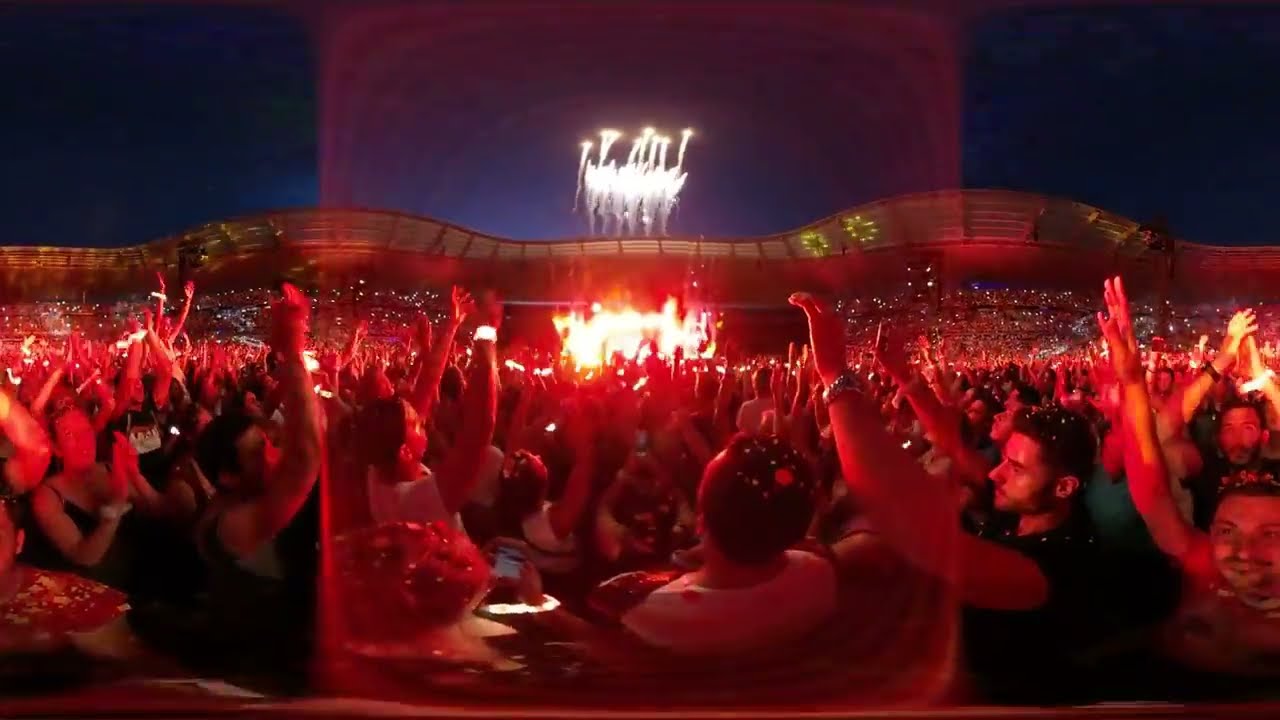The image depicts a colossal outdoor concert, seemingly in a gigantic amphitheater or possibly a sold-out NFL stadium, packed with an immense crowd numbering around 80,000 people. The energetic, electric atmosphere is palpable as attendees raise their hands and numerous cell phones illuminate the scene with their glowing screens. The stage, positioned prominently in the center, is awash in vivid orange, purple, and green lights, making it appear as if it's ablaze. The performance area is so brightly lit that the figures of the band or performers are indistinguishable. Vast crowds, forming mosh pits, are visible scattered across the expansive venue, with people densely packed from the left, center, to the right of the image. Above the stage, the clear, deep blue sky envelops the night, adding to the dramatic backdrop. In the foreground, with enhanced detail, you can spot a man in a white shirt with short brown hair, his back turned to the viewer, and nearby, other concert-goers holding up their phones, their screens shining vividly. The whole scene vividly communicates the exhilarating, buzzing energy of the massive night-time concert.